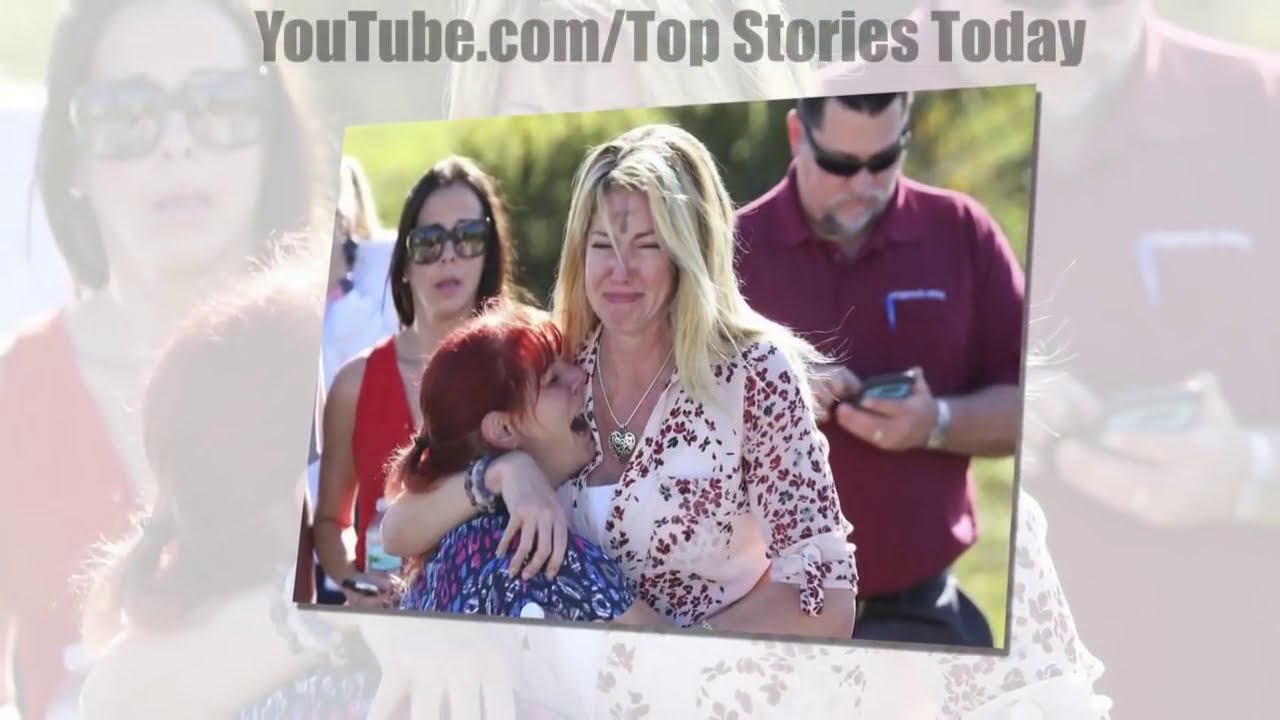This image captures a poignant moment featured on a YouTube channel’s top stories. At the center, a grieving scene unfolds with an older blonde woman, marked with an ash cross on her forehead, dressed in a white top adorned with red flowers, and wearing a silver heart necklace. She holds a younger woman with dyed red hair, who is crying intensely with her mouth wide open, dressed in a blue floral blouse. Surrounding them, in the background, are two other individuals: to the left, a woman in a red top and black sunglasses, also appearing distressed, and to the right, a man with dark hair in a maroon polo shirt, busy on his phone, also sporting sunglasses. The entire image is set against a backdrop that is a zoomed-in, lightened version of the main photo, giving the scene a layered effect. Above this emotional tableau is the gray text: youtube.com/topstoriestoday.